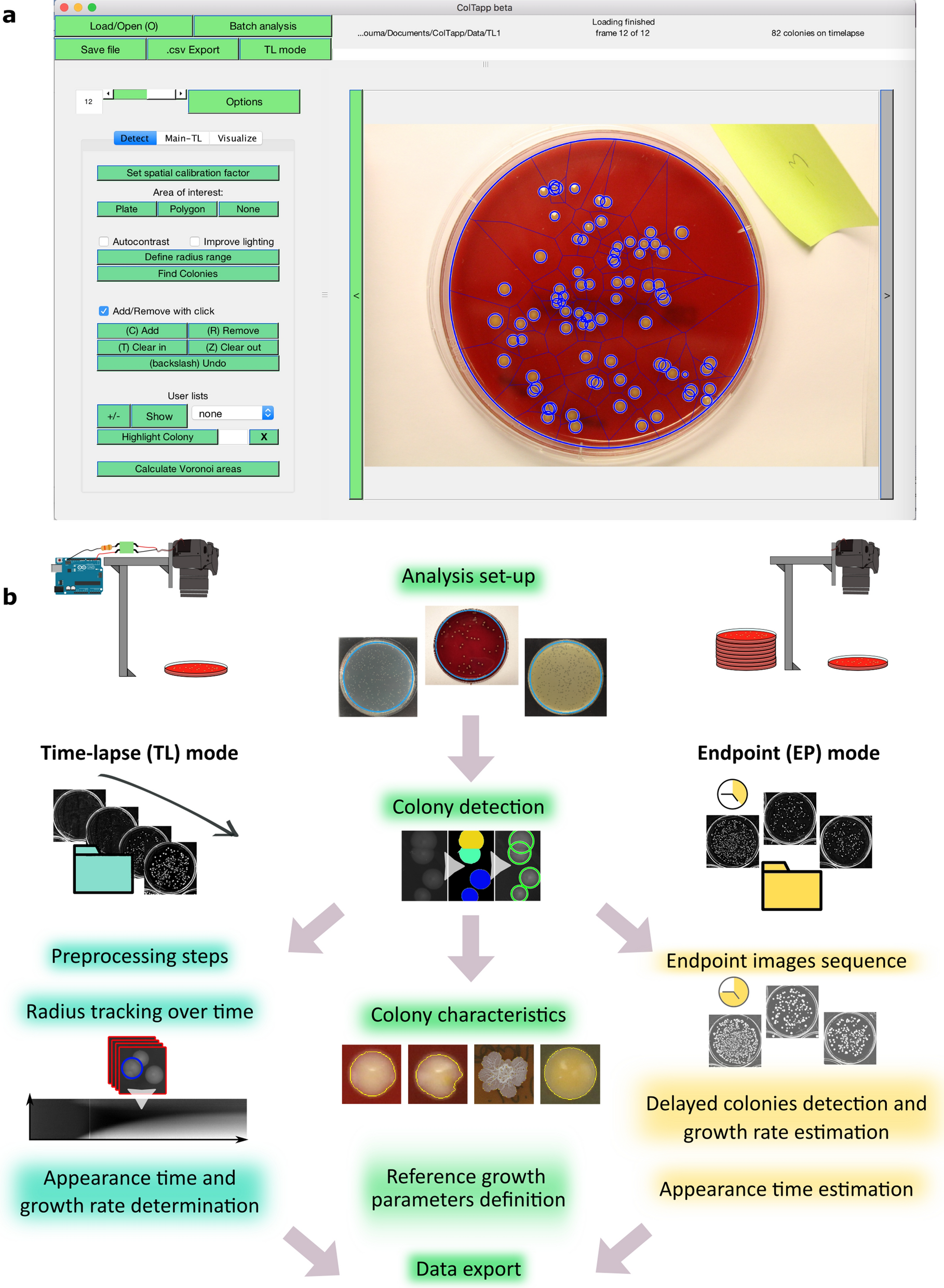This scientific poster meticulously details an experimental process, divided into two main sections labeled A and B. At the top, Section A showcases a computer program interface capturing the analysis of a Petri dish containing red jelly dotted with 35 to 50 purple colonies. The screen capture features multiple actionable tabs such as load open batch analysis, save file, export, and TI mode, alongside various editable fields for data input on the left. Accompanying this digital setup, a small sticky note numbered '3' can be seen on the Petri dish.

Section B is a comprehensive flowchart outlining the experimental procedure and its various stages, illustrated through a series of equipment images and methodological steps. The central pathway includes critical stages like analysis setup, colony detection, colony characteristics evaluation, reference growth parameters definition, and data export. Flanking the top of this nine-image layout are depictions of microscopes observing stacks of Petri dishes. Each procedural step is represented with arrows indicating the order and the diverse outcomes based on the selected pathway. Additional detailed processes include time-lapse mode, endpoint mode, pre-processing steps, radius tracking over time, appearance time and growth rate determination, delayed colony detection, and growth rate estimation. This poster provides an exhaustive guide for laboratory analysts on how to systematically observe and analyze Petri dish colonies, culminating in the efficient export of their data.